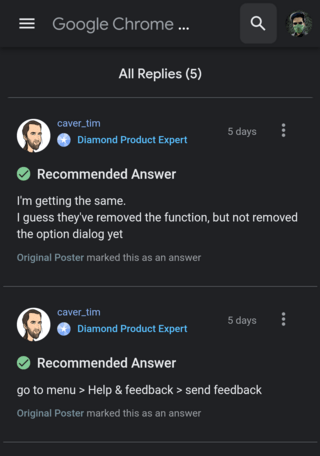This is a screenshot featuring a black background with white and light gray text. In the upper left corner, a menu icon with three horizontal lines is followed by the text "Google Chrome...". Moving to the upper right corner, there is a search icon encompassed by a small box, next to a small circular profile picture of a man who is wearing a green face mask. At the top, the text reads "All replies (5)".

The screenshot displays two replies from a user named "caver_tim", each marked with a blue verification circle featuring a white star in the middle, accompanied by the designation "Diamond Product Expert". To the left of his name, a small circle contains an illustration of his face. The first reply includes a green checkmark followed by the text "Recommended Answer", stating: "I'm getting the same. I guess they've removed the function but not removed the option dialog yet." A second reply from "caver_tim" appears below, also marked as a "Recommended Answer".